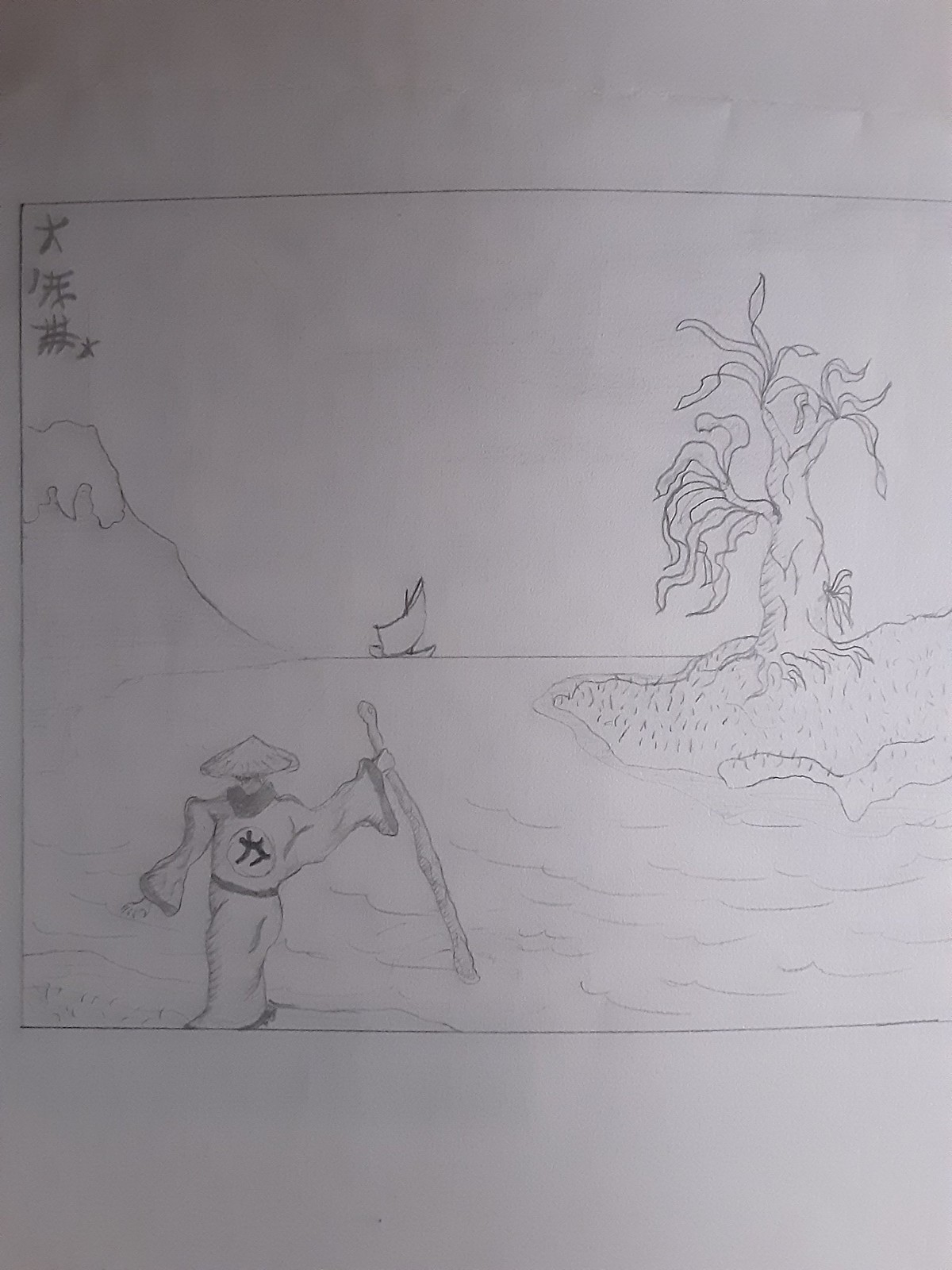This is an image of a detailed pencil drawing on a white sheet of paper, captured in dim lighting that highlights predominantly the right side of the image. Central to the drawing is a square or box-like frame. Within this frame, in the bottom right corner, stands a man dressed in traditional attire, including a long-sleeved robe with a dark belt and a triangular straw hat. He holds a large walking stick or staff and is positioned facing away, looking out over a body of water. His robe features a symbol encased in a circle on the back, indicative of some Japanese or Chinese script.

In the middle of the image, a boat with a single large white sail is visible on the water, seemingly moving from left to right. To the right of the boat, there is a small island with a solitary tree bearing long, slender leaves. On the left side, a prominent snow-capped volcano or mountain descends to meet the horizon line, which marks the boundary of the sea. Additionally, in the upper left of the drawing, there are three vertically oriented Asian characters, possibly Japanese or Chinese, adding further cultural context to the scene. The combination of these elements creates a picturesque and tranquil landscape observed by the robed man.